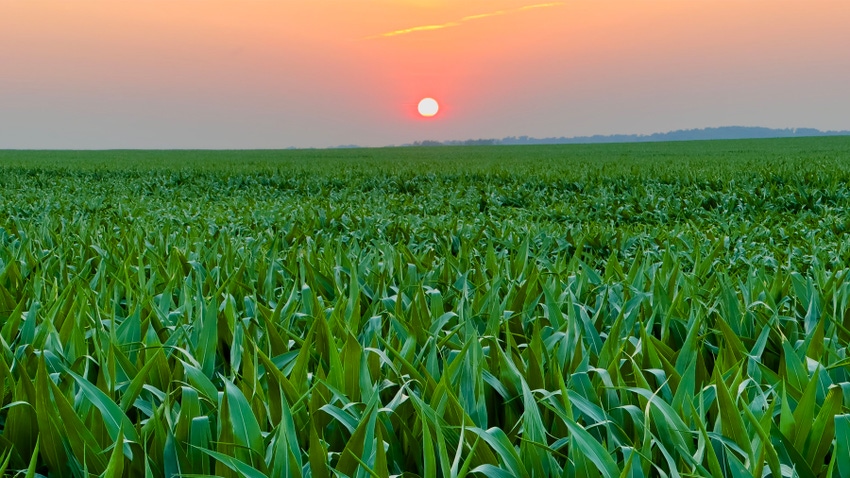The photograph captures a vast agricultural field, likely of corn, stretching out to the horizon. The plants have pointy leaves with light green veins and cover the field entirely. In the distance, towards the right, there is a silhouette of low blue hills or a line of trees. Dominating the upper right of the image is a prominent orange sun, possibly either setting or rising. The sky surrounding the sun transitions through a breathtaking palette; close to the horizon it is a gradient of blue and gray, shifting to vibrant pink, purple, and orange hues as it ascends. A streak of yellow cloud is visible at the top middle of the image. This richly colored outdoor scene, captured during dawn or dusk, highlights the serene beauty of a farm landscape under a captivating sky.